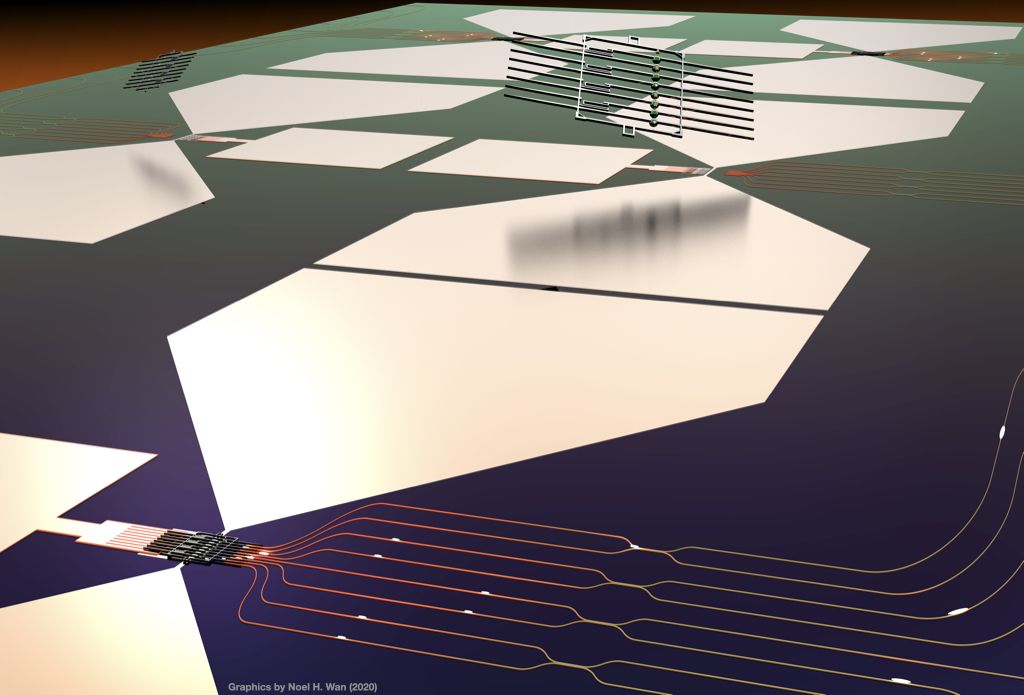The image features an abstract representation of a technological circuit board, possibly a computer chip. The background is a dark, purple-black color, creating a stark contrast against the vibrant elements on the board. Starting from the top, the circuit board displays a gradient of colors transitioning from light green to darker shades of green and purple. Scattered across the board are various geometric shapes—silver, white, and pale pink squares, rectangles, triangles, and other configurations.

Prominently featured is a floating mechanism, consisting of six metal sticks extending from a central square, seemingly suspended in midair. Below this, intricate patterns of electrical lines and electrodes are arranged in an orderly, almost artistic manner; these lines intersect and curve upwards, resembling a network or grid. Several parts of the board include components with glowing red dots and wired connections, lending a dynamic, almost fiber-optic look to the overall design. 

At the bottom of the image, the watermark "Graphics by Noel H. Wan, 2020" suggests that the artwork was created by Noel H. Wan in the year 2020. While the image is rich with various shapes and colors that evoke the internal workings of a piece of technology, it ultimately presents as an abstract drawing, melding elements of electrical circuitry with an artistic flourish.